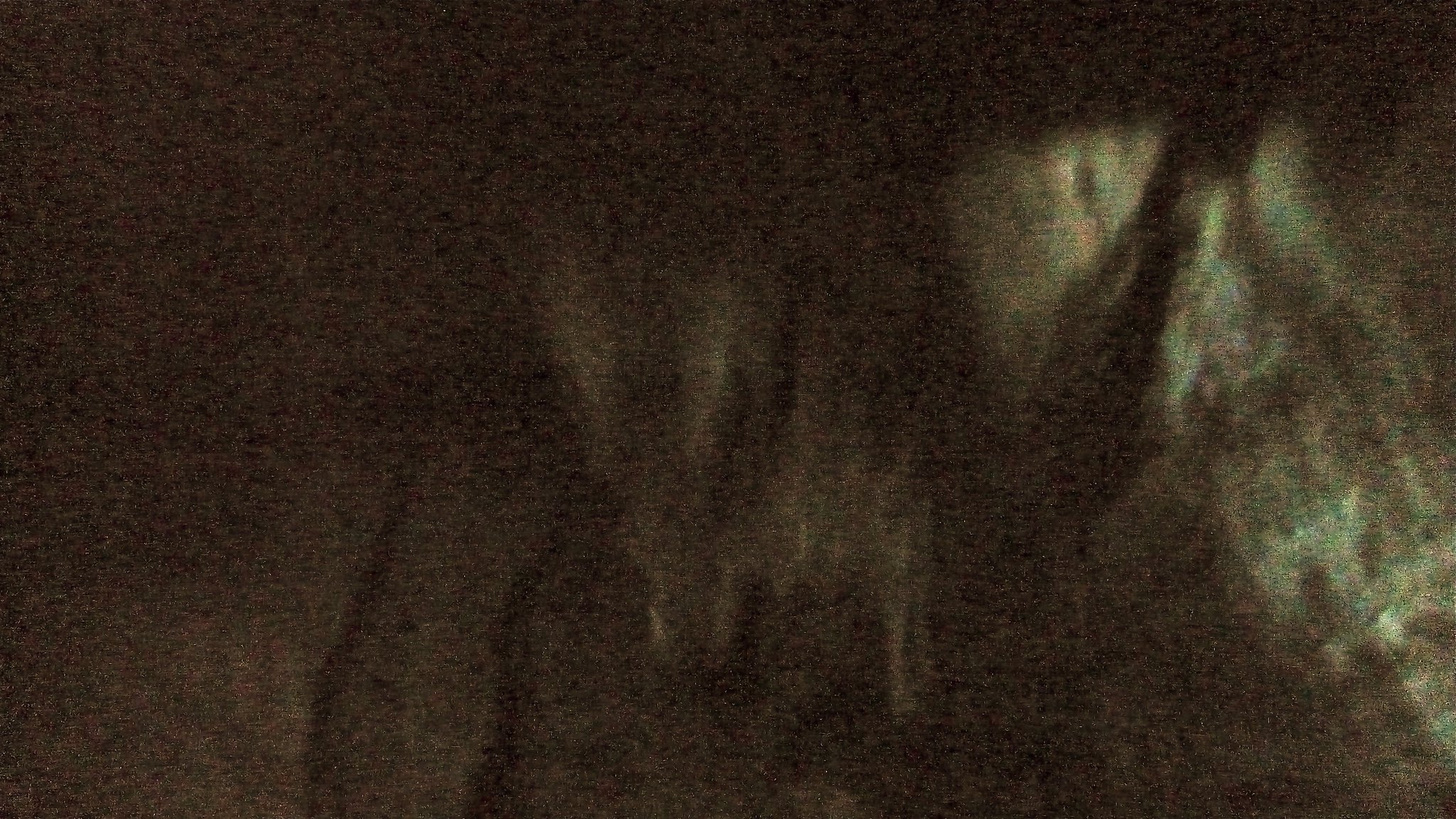The image depicts an extremely blurry and grainy nighttime scene, making it difficult to identify any specific elements. The left side of the image is predominantly dark brown, while the right side exhibits some lighter, yellowish, and greenish hues. There are darker and lighter areas throughout, with the right side being somewhat brighter. An angled streak of darker color runs through the lighter areas. A central shape with distinctive angles and lines of lighter colors can be discerned, but its identity remains unclear. The overall impression is one of a smudged and indistinct composition, suggesting possibilities like a building, trees in a forest, or even abstract patterns, but ultimately defies clear identification.